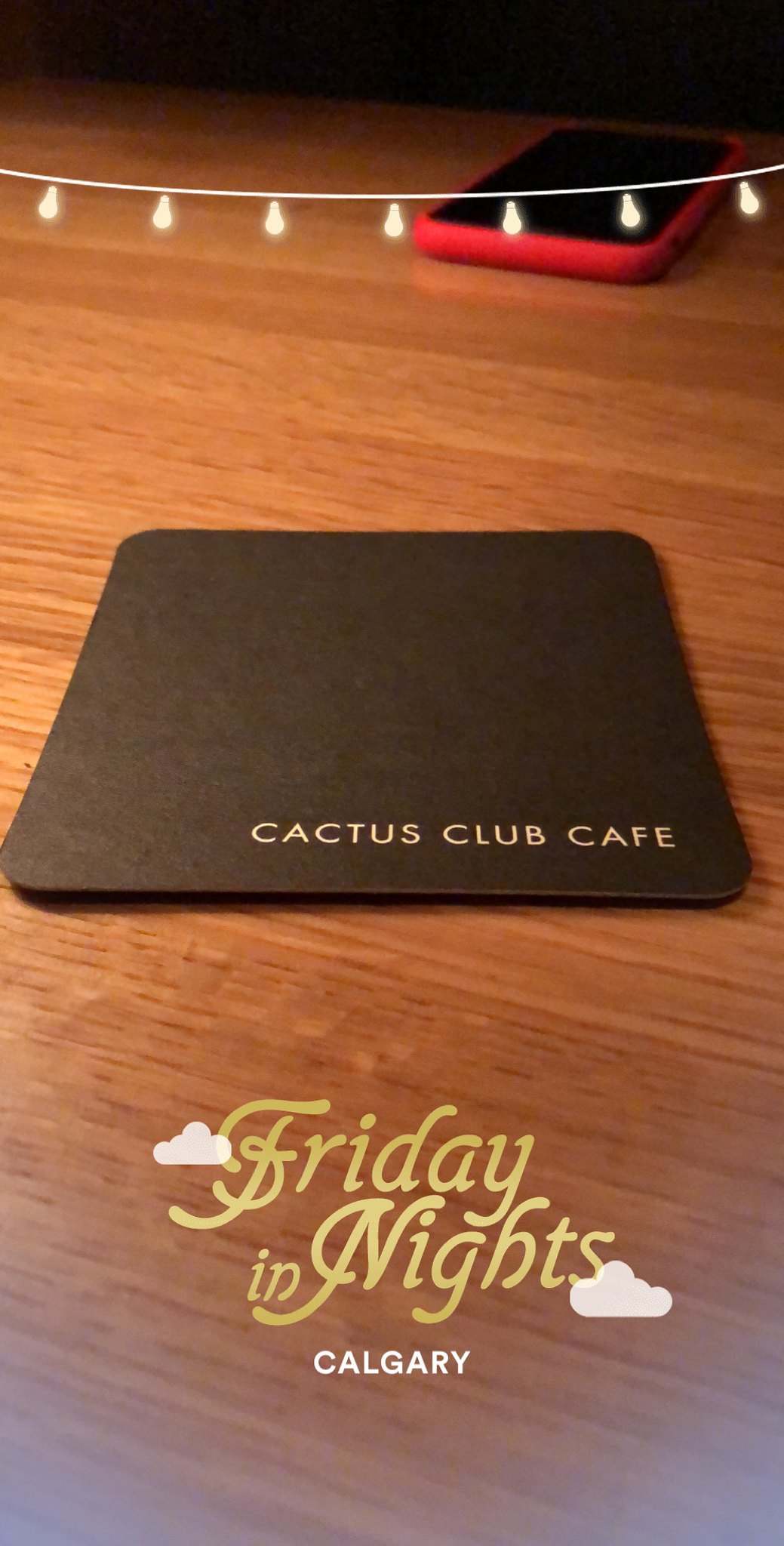The image appears to be a promotional banner or photograph for the Cactus Club Cafe. Dominating the scene is a wooden table upon which a black cardboard coaster with rounded corners is placed. The coaster features gold lettering reading "Cactus Club Cafe". Positioned near the top right of the image is a smartphone encased in red, with its screen turned off. Overlaying the background is a string of seven small fairy lights, contributing to a cozy atmosphere. At the bottom of the image, in an elegant gold font, the words "Friday Nights" are displayed, flanked by small white cloud icons on either side. Below this, the name "CALGARY" is printed in all caps in white. The overall color scheme consists of rich browns, light golden hues, and accents of white and red, with some faded blue appearing at the bottom corners of the image.